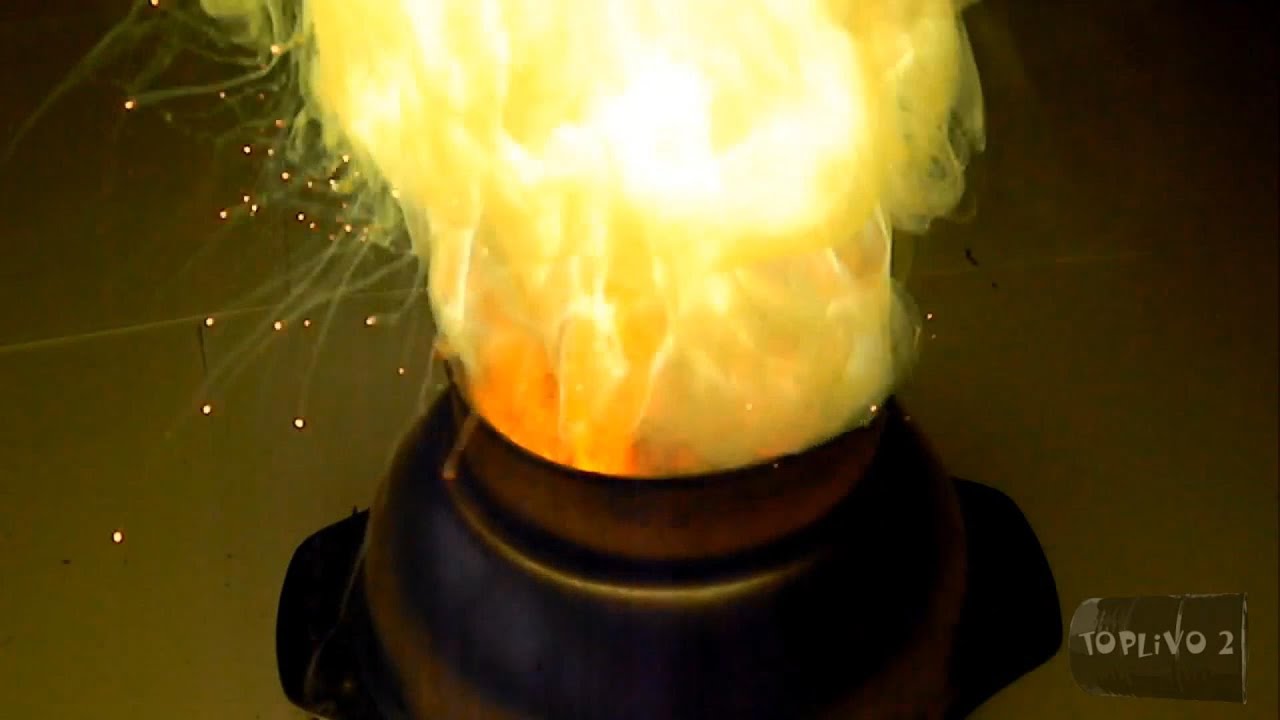The image is a detailed color illustration from a video game, presented in landscape orientation. Dominating the center is a low, round, bronze-colored cauldron set on a dark, handled platter. A fiery explosion of smoke and flames erupts from the cauldron's top, with the flames transitioning from intense orange near the cauldron's mouth to a bright yellow and white mix higher up. Sparks fly off towards the left side amidst flumes of smoke that vary from yellow to white. The background is a deep, dark brown, which contrasts sharply with the vivid, bright light at the center of the flames. In the bottom right corner, there's a small, beige-toned tag-shaped object with text that appears to read "Top Live-O 2." The overall style and composition suggest that this is a video game illustration.